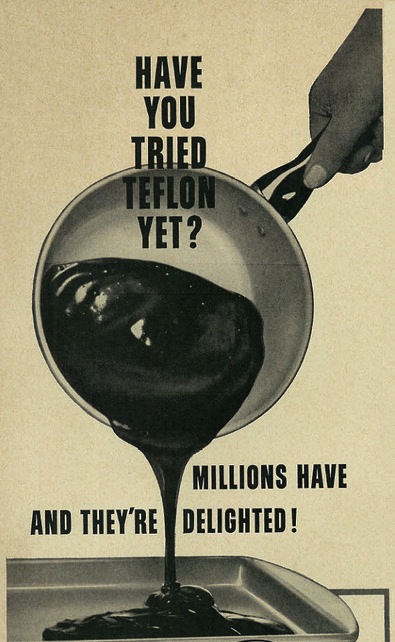This vintage, black-and-white advertisement from the 50s or 60s, displays a yellowed poster with bold black letters that read, "Have you tried Teflon yet? Millions have and they're delighted." The central image features a manicured hand in the upper right-hand corner, holding a shiny, metallic saucepan with a sleek black handle. Inside the pan, a shiny, dark liquid—possibly a chocolate sauce or brownie batter—drips smoothly down into a metal baking sheet below, emphasizing the stick-free quality of Teflon. The background and objects maintain a classic, monochrome aesthetic typical of mid-20th-century advertising.